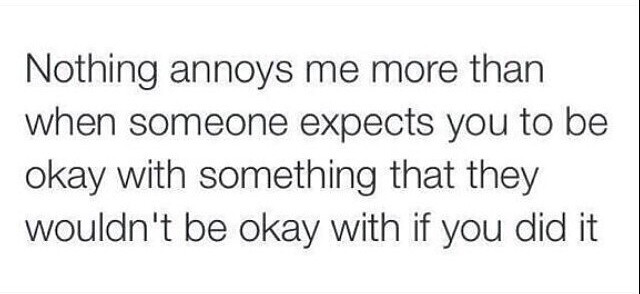The image showcases a simple, white backdrop with black, thin text that reads: "Nothing annoys me more than when someone expects you to be okay with something that they wouldn't be okay with if you did it." The lettering starts with a capital "N" for "Nothing" while the rest of the text remains in lowercase without any punctuation marks. The height of the letters is approximately 1 1/2 inches. Additionally, there is a long black line parallel to the text on the right-hand side, measuring around three inches. The overall composition is minimalistic and clear, emphasizing the message conveyed by the text.